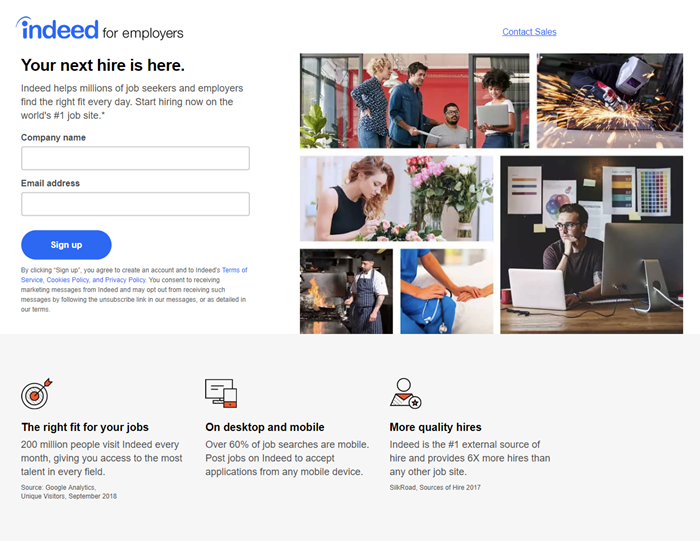Screen capture from the Indeed employment website: In the upper left corner, the Indeed logo is prominently displayed, followed by the word "Indeed" in blue text, designed for employers. Adjacent to the logo, the header reads, "Your next hire is here." Below this, there are fillable sections labeled for "Company Name" and "Email Address," followed by a "Sign Up" button.

To the right, a vibrant collage showcases a variety of professional settings: the upper left corner features an office environment, while the upper right highlights a welder at work. The lower right depicts an individual at a desk, the lower left captures a chef in action, and another image portrays a nurse bedside. 

At the bottom of the page, three informative columns are presented. The left column, titled "The right fit for your jobs" in bold black, includes a bullseye with an arrow icon above it. The middle column, labeled "On desktop and mobile" in bold, is placed alongside an appropriate icon. The rightmost column, entitled "More quality hires," also features a corresponding icon. Each column contains a brief, one-sentence blurb beneath its header.

Overall, the webpage is designed to assist employers in signing in and setting up their accounts to use Indeed for finding prospective hires. The colorful images to the right predominantly depict professionals engaged in various work environments, aligning with the theme of recruitment across diverse industries.